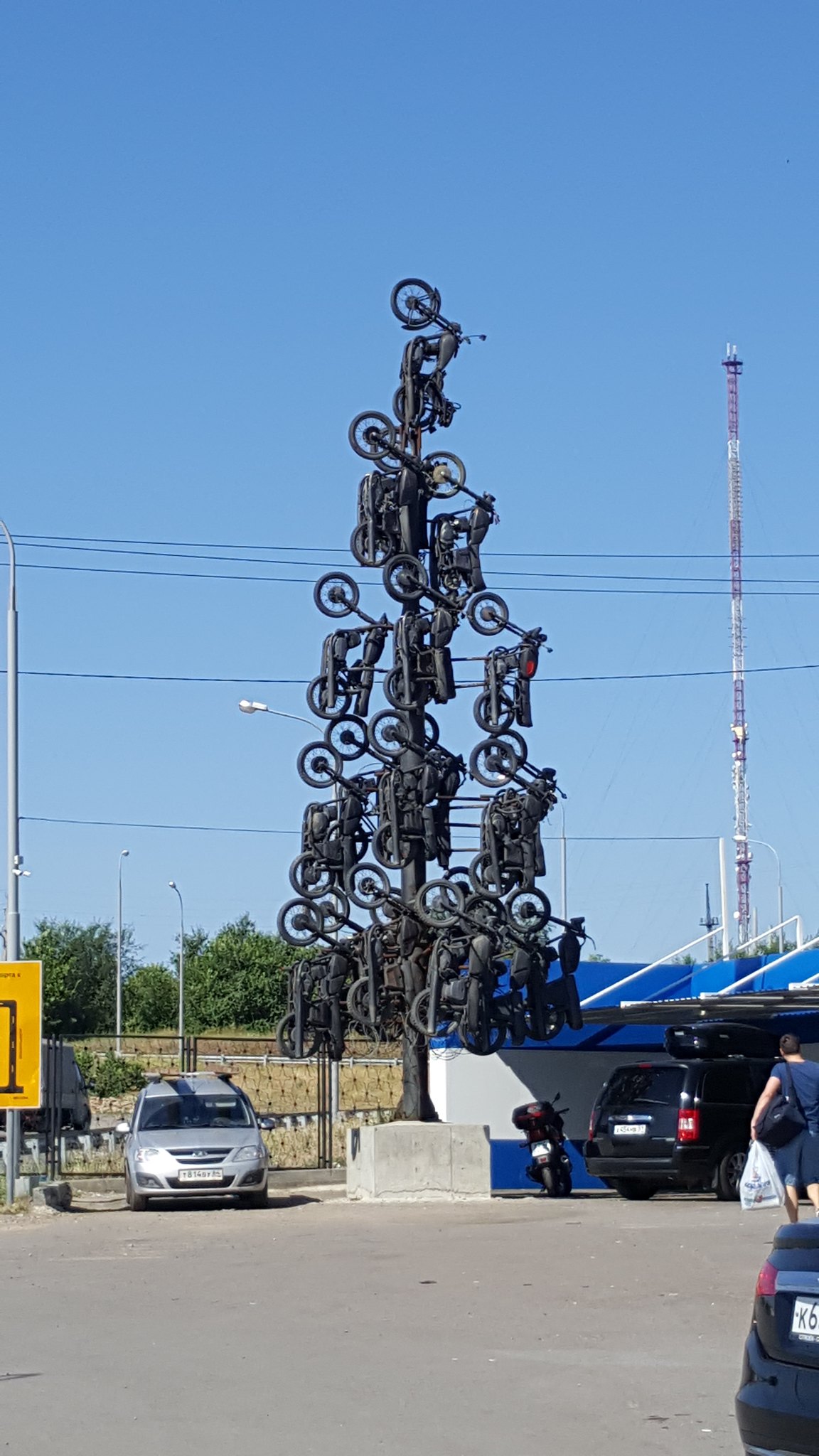The photograph depicts an outdoor scene centered around an impressive, artistic sculpture. The sculpture, composed of black-painted motorcycles, takes on the shape of a Christmas tree, with a wider base tapering off towards the top. The motorcycles are real, all the same make and model, and arranged in layers: approximately ten at the base, diminishing to a single motorcycle at the peak, rising to about three or four stories high. They are mounted on a square cement base, with a central pole supporting the structure. Notably, one motorcycle sports a red seat, adding a touch of contrast to the otherwise monochromatic display.

Surrounding the sculpture, the environment suggests an urban setting with a concrete surface, resembling a parking lot. A gray car is parked to the left of the statue, and several other vehicles are visible in the lot. A blue sky with some green trees can be seen in the background, along with a white building featuring a blue stripe and roof. 

To the right of the sculpture stands a woman, identifiable by her blue top and shorts, carrying a white grocery bag and a blue purse. Behind her, a red and white cell phone tower and multiple electrical lines are visible, adding to the intricate backdrop. Additionally, a yellow sign peeks out from the left side of the scene. This detailed composition blends modern art with urban life, capturing a unique and engaging moment.